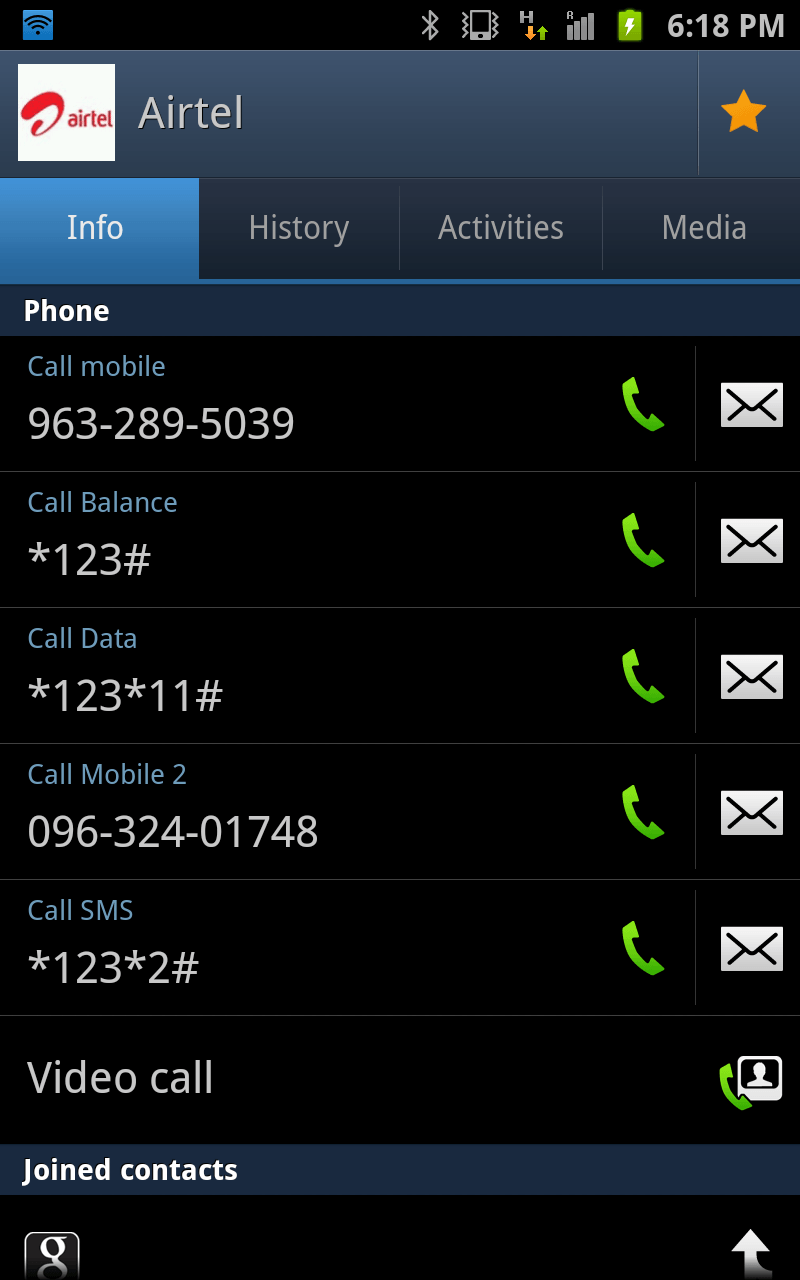A detailed, cleaned-up caption for the image could be:

"A screenshot of an active cell phone screen displaying the Airtel network on the top left corner, marked with a white font and accompanied by a red swirl logo in a white box. The screen shows several tabs labeled 'Info,' 'History,' 'Activities,' and 'Media' in white font below the Airtel identifier. The 'Info' tab is highlighted with a light blue background, indicating it is currently selected. Below these tabs, there is a section titled 'Phone' which lists five call entries. These entries include details such as 'Call Mobile' with a phone number, 'Call Balance,' and 'Call SMS,' each written sequentially. The display is characterized by a minimalist design with clear, readable text and organized sections for easy navigation."